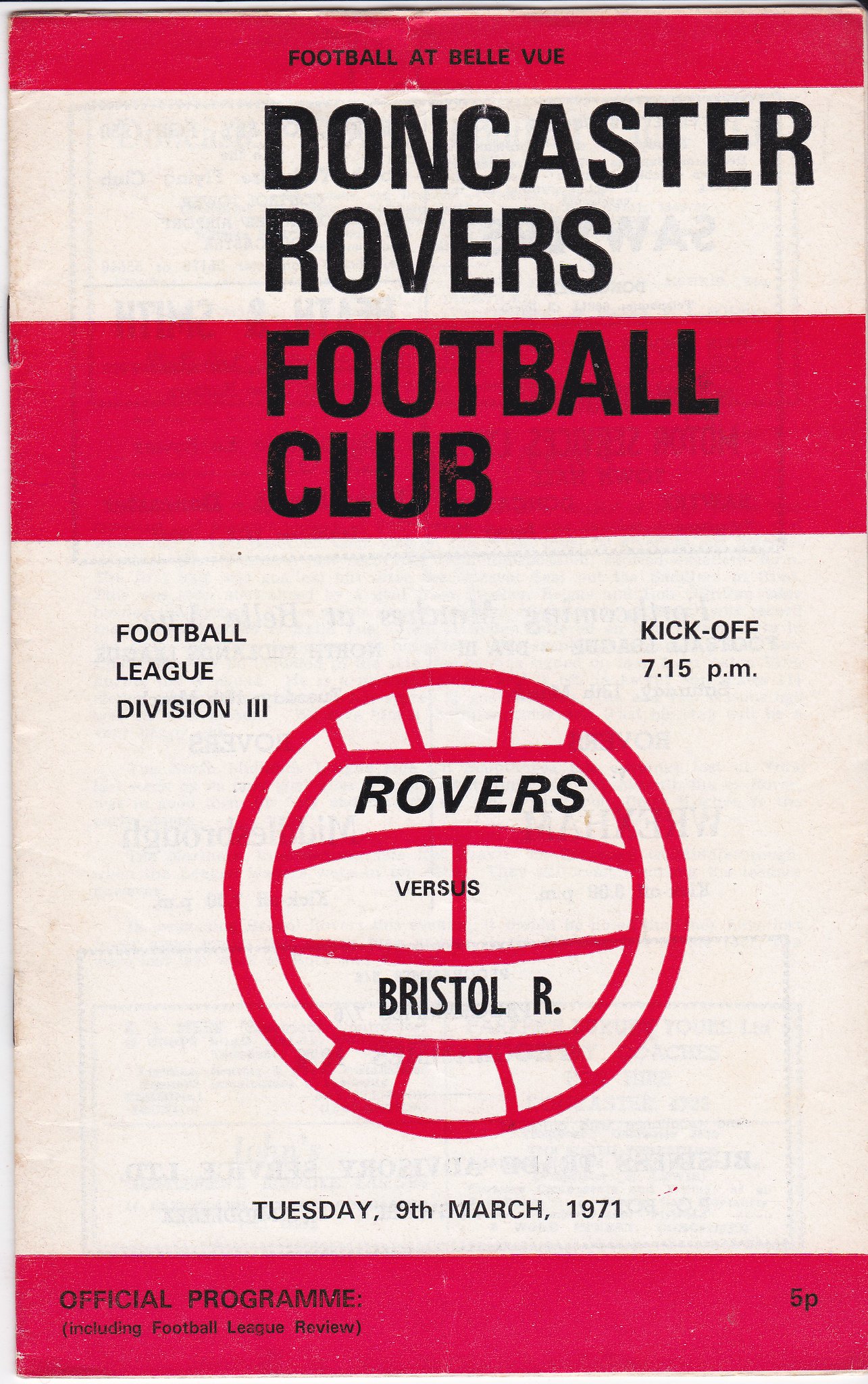This image features the cover of the official program for the Doncaster Rovers Football Club's match against Bristol Rovers, dated Tuesday, 9th March 1971. The design indicates it is from the 1970s, with aged and slightly faded colors. The program cover prominently showcases a red and off-white color scheme with black text. At the very top, a red banner with the text "Football at Bellevue" in black is followed by a white section that says "Doncaster Rovers" and then another red section stating "Football Club." Centered on the cover is a simple, crude line drawing of a soccer ball, with the match details contained within and around it. Inside the ball, it reads "Rovers versus Bristol R." To the right of the ball, the text states "Kickoff 7:15 p.m.," and to the left, it says "Football League Division Three." Below the ball, the date is specified as "Tuesday, 9th March 1971." The bottom of the program features another red stripe where the left side announces "Official Program (including Football League Review)" and the right bottom corner mentions "5p." The overall design hints at its vintage nature and its purpose as an official matchday program.